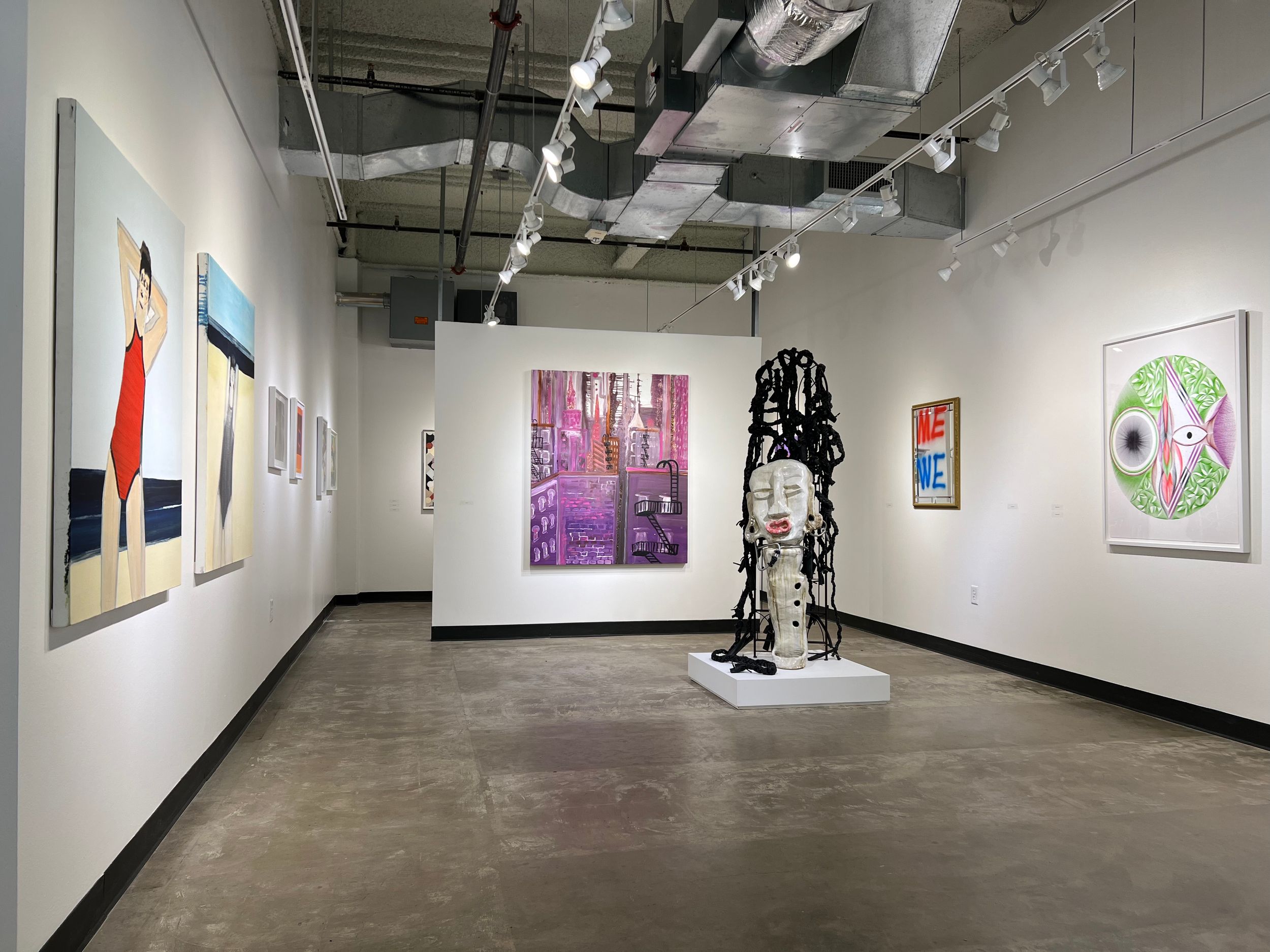This image captures an art gallery exhibition with stark white walls and a concrete floor illuminated by industrial showroom lights and exposed HVAC ducts on the ceiling. Centrally positioned in the gallery is a striking sculpture of a woman's head, notable for its hyper-realistic, oversized features, including pronounced red lips, a wide nose, and closed eyes, crowned with intricately sculpted black hair. Framed by a black gauze-like material, the sculpture evokes a sense of enigmatic presence. Surrounding this central fixture, various artworks are displayed: a painting featuring a cityscape with bricks and a black fire escape ladder, a colorful "Me We" text art framed in red and blue, and a portrait of a woman in a swimsuit standing by the water. Additional varied, abstract artworks in vibrant hues of orange, red, blue, green, and purple fill the walls, contributing to a dynamic and engaging visual experience. The overall ambience of the gallery is both modern and industrial, highlighted by meticulous lighting that accentuates each piece on display.